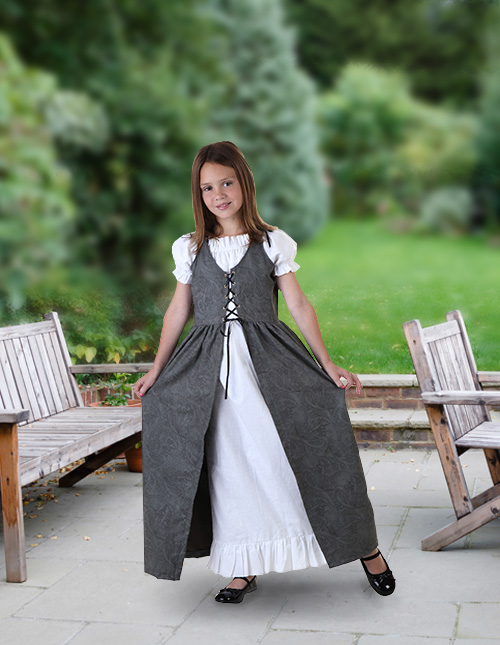The photograph is a vertically rectangular, color image taken outdoors in natural daylight. It features a staged scene with a cute young Caucasian girl who has shoulder-length brown hair and a pleasant smile. The background, which occupies the top two-thirds of the image, is a lush, green blur of grass, bushes, and trees, including a noticeable pine tree. The setting is a stone patio in a backyard, featuring wooden furniture—a rocking chair positioned to the center-right and a bench to the center-left.

The girl is the focal point of the picture. She is dressed in a charming outfit that resembles traditional peasant or Amish attire. Her ensemble includes a white, fitted bodice that transitions into an A-line dress with ruffled sleeves and hem. Over this, she wears a dark gray, peasant-style overlay that features a buttoned bodice and opens into a V-shape below the bodice, revealing the white dress underneath. She is holding out the split sections of the gray overlay, as if in a curtsy, showcasing the detail of both garments. She completes her outfit with flat black strap shoes that buckle around her ankles. The overall scene is idyllic and beautifully captures the girl proudly modeling her distinctive, charming attire.